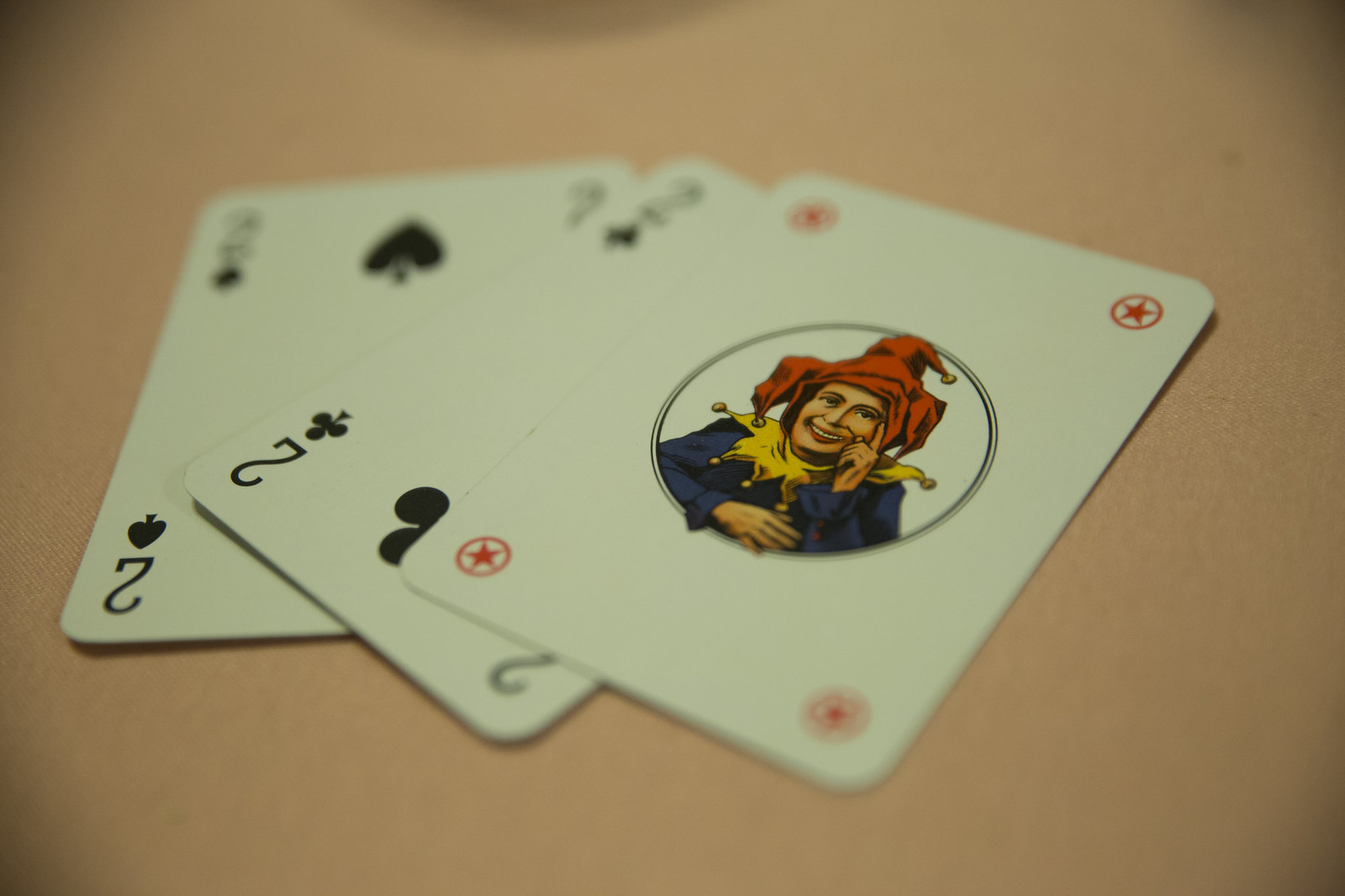This close-up photograph captures three playing cards artistically arranged on a beige tablecloth surface. The cards are slightly overlapping, and from bottom to top, they display a Two of Spades, a Two of Clubs, and a Joker. Each card features a white face with distinct designs.

The Two of Spades, positioned at the bottom, showcases a bold black '2' and a spade symbol—a heart with a short, downward-pointing stem. Above it is the Two of Clubs, which mirrors the black '2' and introduces a club symbol resembling a trio of black circles forming a triangle atop a small base.

Dominating the topmost position, the Joker card is richly adorned. Each corner is marked by small red stars encased within circles. Central to the card is a larger, double-outlined circle housing the jovial face of a jester. This figure is grinning broadly, donning a vibrant red hat with yellow bells, a pointed yellow collar also jingling with bells, and a blue long-sleeve top. The jester's playful demeanor is accentuated by his hand gestures, with one hand resting gently beside his face and the other poised in front of his chest.